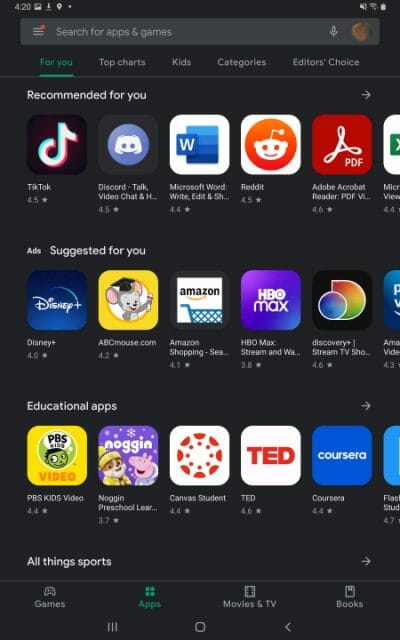The image displays a smartphone screen showing a user navigating an app store. At the top of the screen is a search menu that allows the user to look for apps and games. Below the search menu, a series of menu tabs stretch across the screen, including "For You," "Top Charts," "Kids," "Categories," and "Editor's Choice." The "For You" tab is currently selected, indicated by its green highlight.

Beneath the menu tabs is a section titled "Recommended for You," showcasing a selection of app icons such as TikTok, Discord, Microsoft Word, Writer, Reddit, and Adobe Acrobat Reader. Following this is an ad section named "Suggested for You," featuring apps like Disney, ABC Mouse, Amazon Shopping, HBO Max, and Discovery Stream.

Continuing downward, there is a section for educational apps, displaying icons for PBS Kids Video, Noggin's Preschool, Canvas Student, TED, and Coursera. Additionally, there is an "All Other Sports" section mentioned, however, it requires scrolling to view its contents.

At the very bottom of the screen, there are navigation icons for "Games," "Apps," "Movies & TV," and "Books." The "Apps" icon is currently selected.